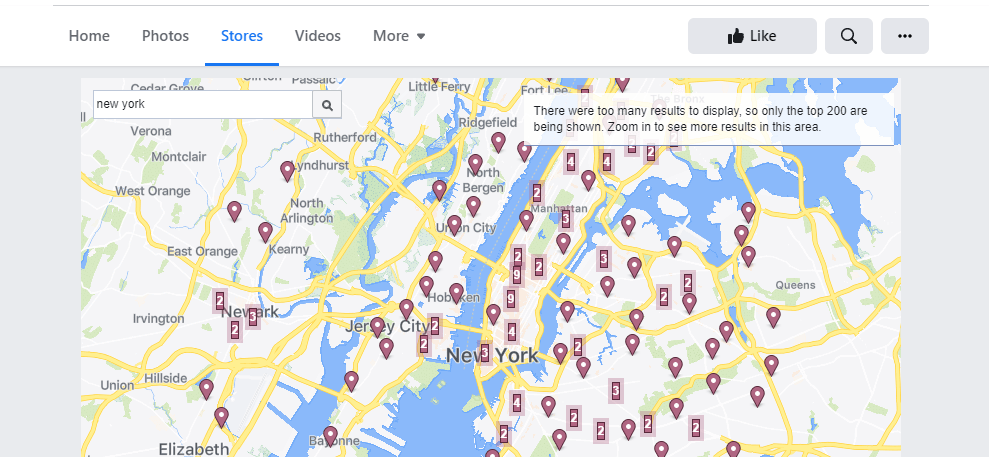The image is a detailed screenshot set against a white background with a light gray border at the top. At the upper section, there are navigational tabs including "Home," "Photos," "Stores" (which is highlighted in blue and underlined), "Videos," and a "More" dropdown option. In the upper right corner, there are icons for liking (thumbs up) and a magnifying glass for search.

Below the tabs is a large, expansive map that stretches from the left to the right side of the image. This map features numerous red pins and red rectangles, with a high concentration of these pins located in New York. Notable areas on the map include Queens on the east side, and Manhattan to the west, both densely covered with red pins indicating various locations. The roads are clearly outlined in yellow, while the ground and surrounding areas are predominantly white with occasional green patches. The map also highlights the peripheral river encircling Manhattan in a distinct blue color.

To the left side of the map, New Jersey is depicted, showcasing multiple pins in specific areas such as Jersey City, Hoboken, Union City, North Bergen, Ridgefield, and Fort Lee. Additionally, there are a few scattered pins in the East Orange region. This visual representation emphasizes the dense clustering of points of interest around major urban zones.